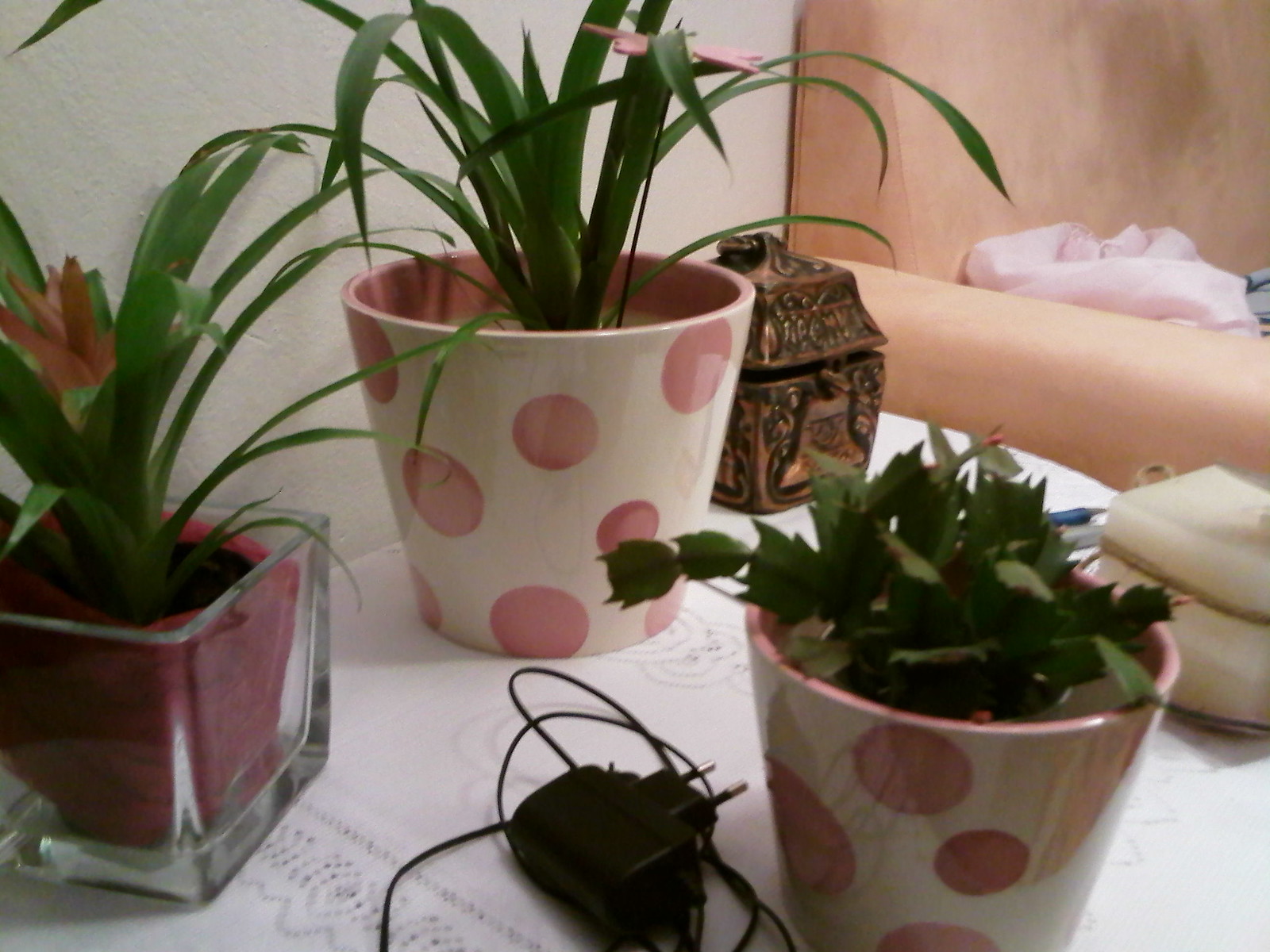This amateur photograph captures a cozy domestic scene featuring a collection of houseplants arranged on a side table next to either a couch or a bed. The table is draped with a white lace tablecloth, adding a delicate touch to the setting. Prominently displayed are two plants in white pots decorated with pink polka dots, each sprouting tall, grass-like greenery. Adjacent to them is a third plant housed in a cubic, transparent glass vase, which contains another pink planter inside it. The table also holds a UK plug charger cord and a small, indiscernible corporate trinket on the far left. Behind this verdant display, a metal box and another indistinct object are partially visible. The background reveals a corner of a sofa or chair adorned with a pink throw, completing the homely atmosphere of the photograph.